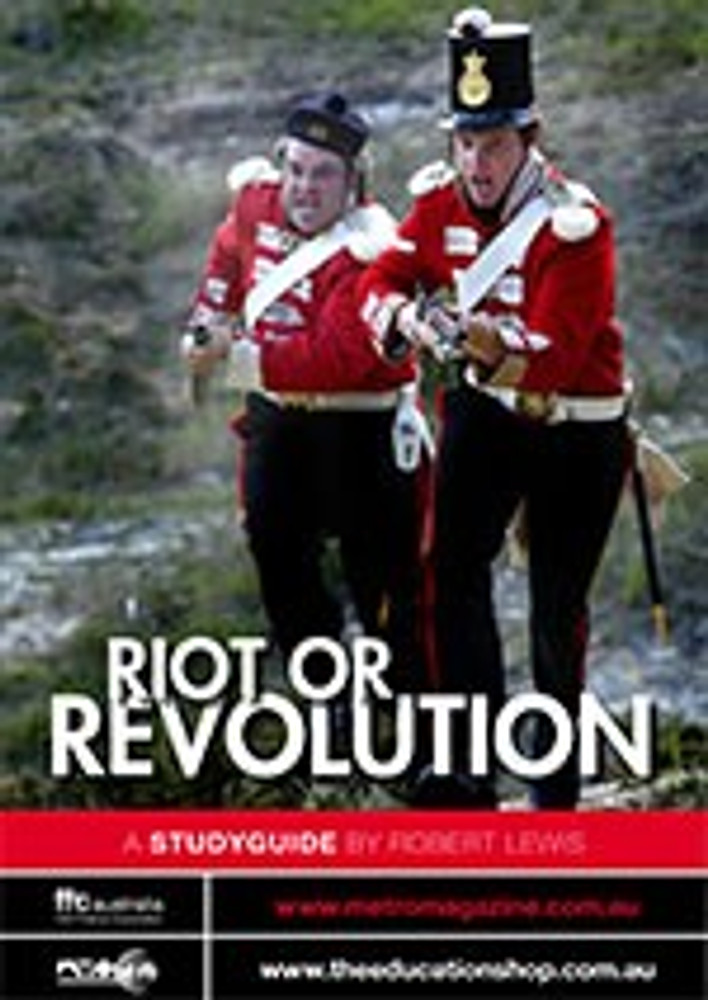The image is a detailed, promotional movie poster or study guide cover titled "Riot or Revolution" by Robert Lewis. It features two British soldiers from the Revolutionary War era, dressed in distinctive red coats with white sashes and shoulder pads. Both soldiers are depicted running towards the viewer with menacing expressions and pointed rifles, as if ready to engage in a bayonet charge. The soldier in the foreground is thinner and wears a tall black hat adorned with a feather and a gold medallion, while the heavier-set soldier in the background sports a dark blue beret. Both soldiers carry swords at their sides, black pants with red stripes, and white belts with gold buckles. They are shown charging over a grassy and patchy terrain. The title "Riot or Revolution" is prominently displayed in white text at the bottom of the poster, and above it, in red text on a white background, reads "A Study Guide by Robert Lewis." The bottom of the poster also hints at a website, though it is partially unreadable.